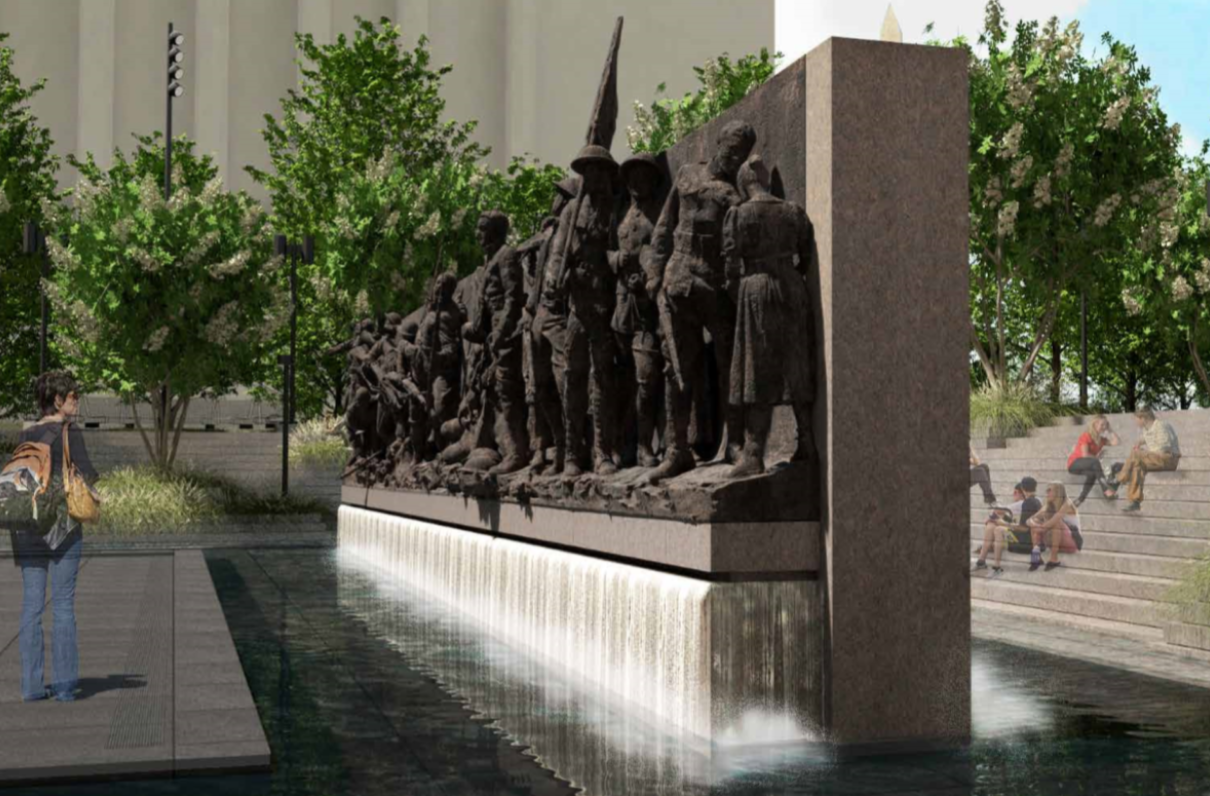The photograph depicts an outdoor commemorative monument that seems to blend reality with artistic surrealism. This large granite structure features an intricately carved scene of soldiers, some carrying flags and wearing hats, with a woman in a dress standing prominently in the foreground. A waterfall cascades down from a ledge into a large square pool at the monument's base, creating a serene watery tableau. White crepe myrtles in bloom frame the background, enhancing the scene's tranquility. On the right, granite steps host several tourists, about six, who oddly appear translucent, giving them a ghostly or holographic appearance. On the left, a person in jeans with a backpack gazes at the monument, also possessing this eerie transparency. The backdrop includes a large white building, potentially suggesting a location in Washington, D.C. This unconventional mix of realistic details and holographic imagery creates a mysterious, almost ethereal atmosphere around the monument.